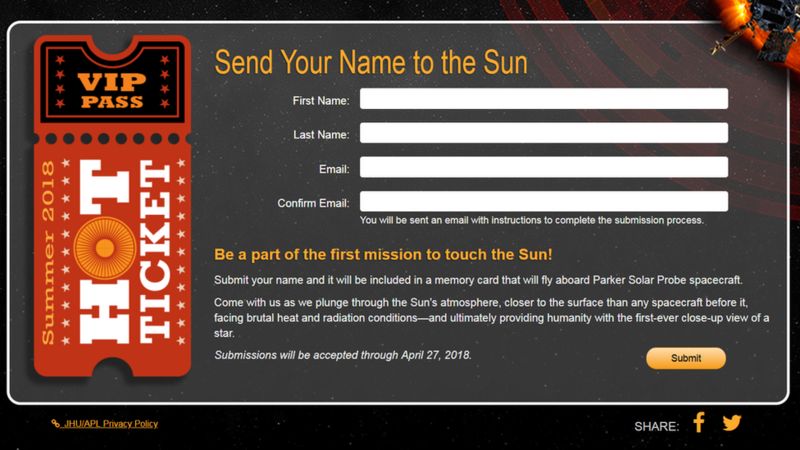A website screenshot features a VIP pass for a special event. At the top of the ticket, "VIP" is prominently displayed in large, bold orange capital letters, followed by the word "PASS" in smaller, yet still capitalized letters. Just below this heading, in orange print, the text "Summer 2018" is visible. Adorning the ticket are star icons and the phrase "HOT TICKET," where the "H" and "T" are capitalized in white, and the "O" is artistically designed to resemble a Ferris wheel in an orange hue.

Above the ticket, the webpage header invites visitors with the message "Send Your Name to the Sun." Instructions followed by white text boxes request user details: the first box for a first name, the second for a last name, the third for an email address, and a fourth for email confirmation. Below these fields, an orange text encourages participation in a historic space mission. It reads, "Be a part of the first mission to touch the Sun. Submit your name, and it will be included in a memory card that will fly aboard Parker Solar Probe spacecraft." A submit button is also visible at the bottom.